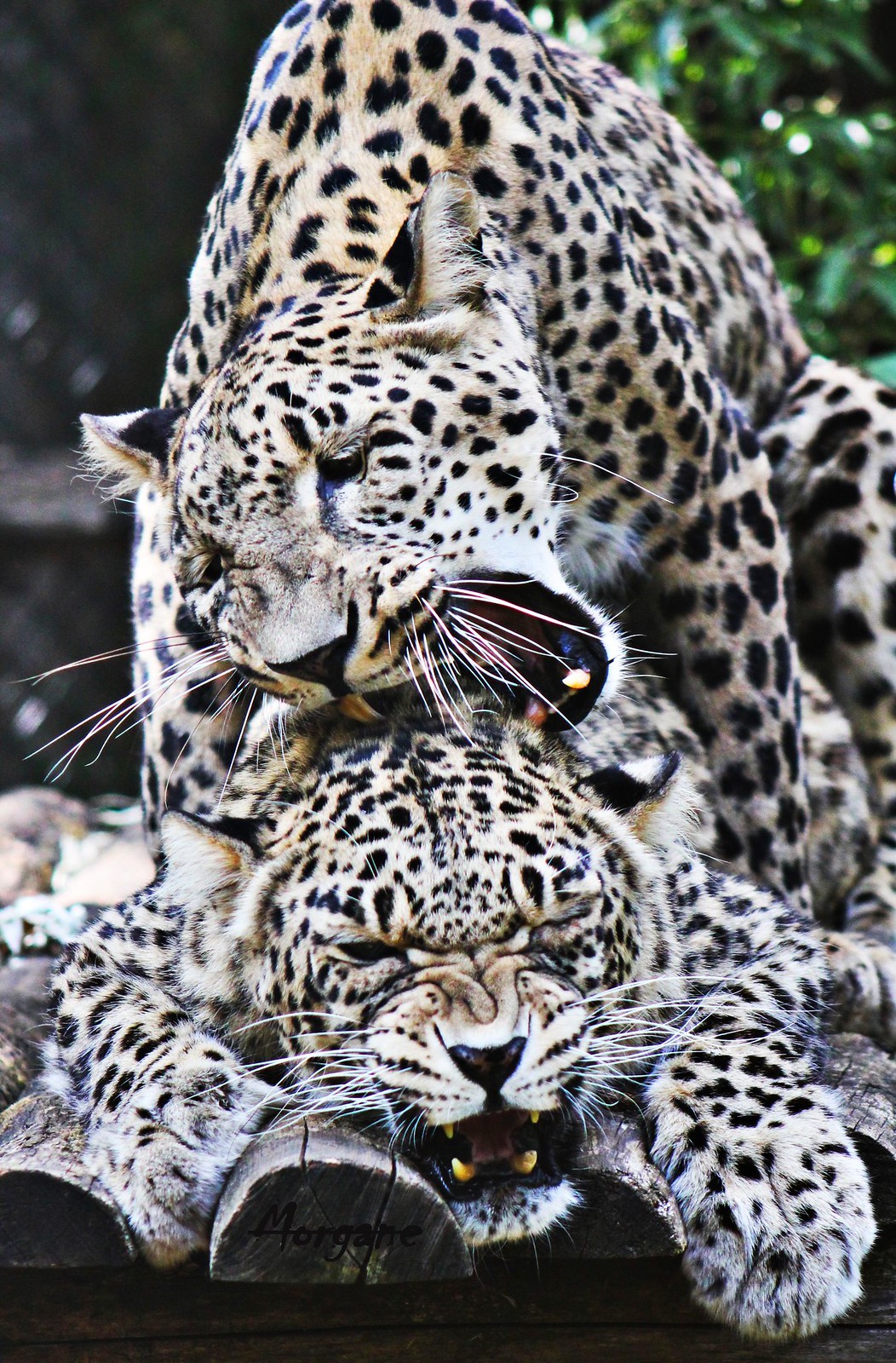In this outdoor photograph, likely taken in captivity due to the presence of man-made structures, two large, speckled felines—appear to be leopards—are captured in a dynamic, possibly aggressive or mating pose. The leopard on top is mounting the other, with its mouth open and gripping the back of the neck of the one beneath. The lower leopard is lying flat on a wooden platform constructed of several aligned small logs, with its front paws visible and its mouth open in an expression that could indicate pain or annoyance. The background shows a glimpse of greenery, suggesting a tree within the enclosure, and possibly a blurred fence. Notably, the photograph includes the name "Morgane" printed on it, indicating the photographer’s name.